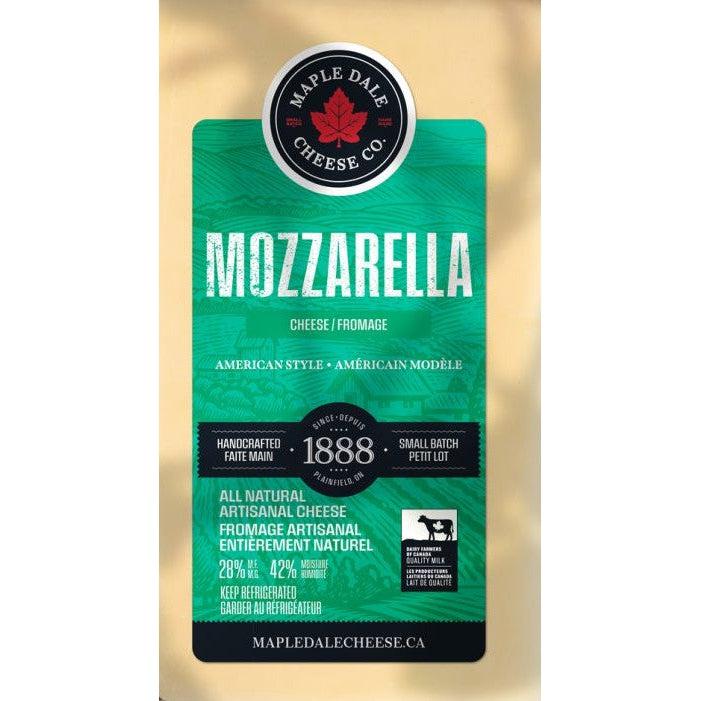This detailed photograph captures the packaging of a handcrafted, artisanal mozzarella cheese by Maple Dale Cheese Co. The layout is in portrait format, featuring a prominent green label with rounded corners set against a cream-colored background, resembling the cheese itself. At the top of the label, there is a distinctive logo comprising three concentric circles—white, black, and thin white—with a red maple leaf centered in the black circle. The text "Maple Dale Cheese Co." encircles the leaf.

The central green label features white capital letters spelling "MOZZARELLA," followed by "CHEESE / FROMAGE," and "AMERICAN STYLE / AMERICAN MODEL." Below this is a black bar inscribed with "Handcrafted / Fait à Maine / 1888 / Small Batch / Petite Lot" in white text. The green background resumes, detailing the cheese as "All Natural / Artisanal Cheese / Fromage Artisanal / Entertainment Natural," and specifying "%28" and "%42" ingredient percentages. It also advises "Keep Refrigerated," with the French translation included.

On the right side of the label, there is a black and white logo featuring a cow, and just below this is another black bar with white text reading "MapleDaleCheese.ca." In the background of the green label are subtle impressions of a farm scene with rolling hills, enhancing the product's artisanal and natural appeal.